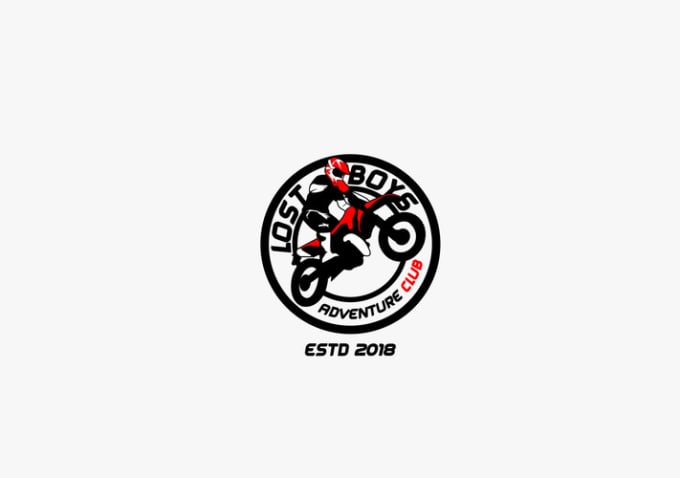The image features a rectangular logo approximately 5 inches wide by 3 inches high, with a faint light gray background. At the center of this rectangular space is a round emblem containing two concentric circles. A motorcyclist on a red dirt bike, which has black wheels and handles, is depicted in mid-jump, pulling the front wheel higher than the back, and standing upright on the bike. The rider wears a red and white full-faced helmet, a black and white suit, and matching black and white motocross boots. The outer circle of the emblem contains the text "Lost Boys Adventure Club" in black at the top, with "Club" highlighted in red. Below the circles, it reads "ESTD 2018" in bold black print, indicating that the Lost Boys Adventure Club was established in 2018.